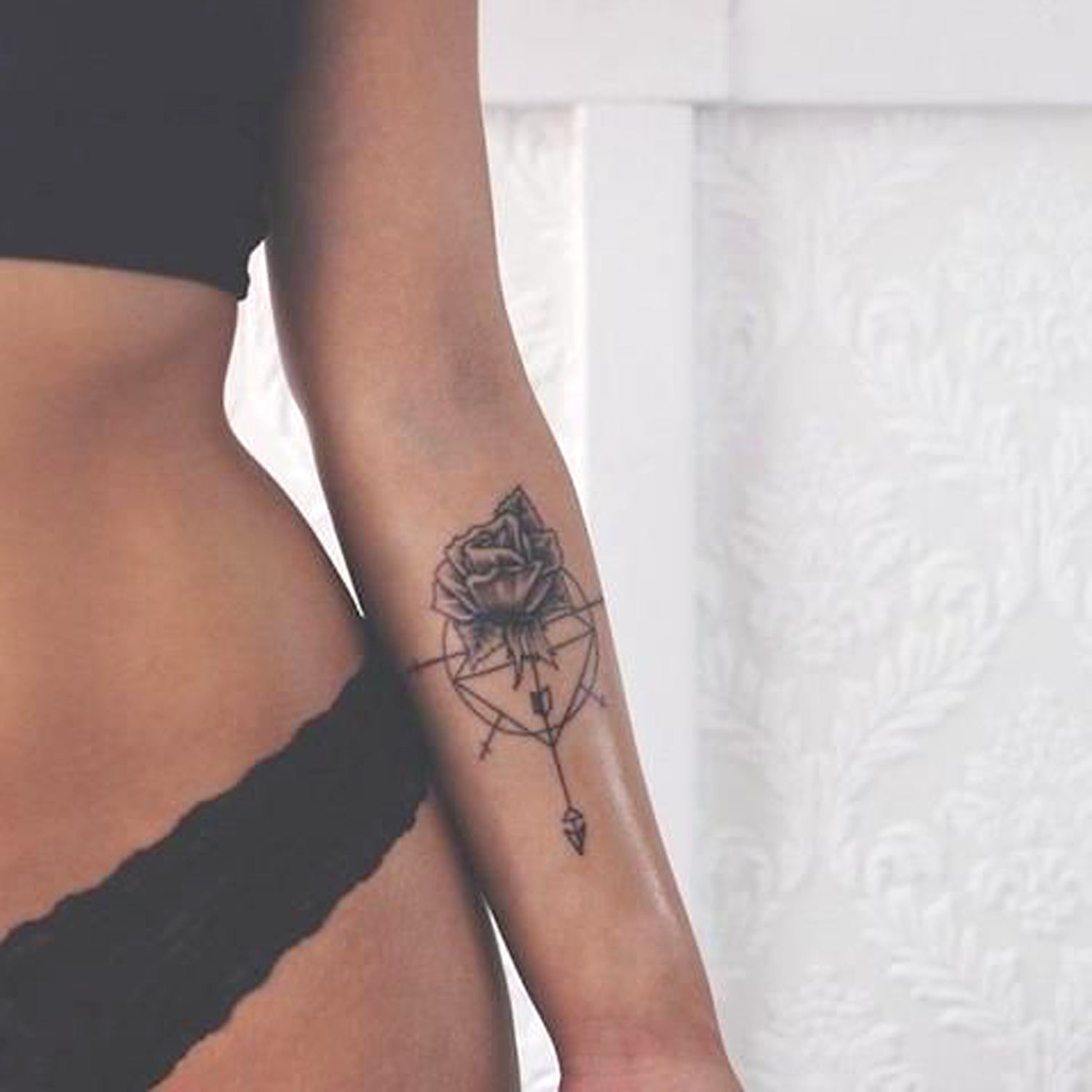This photograph captures a detailed view of a woman from her chest to her hips. Her skin is a tan, brown shade, and she is wearing a black bra and black underwear. The focus is on her left forearm, which features a striking black-and-gray tattoo. The intricate tattoo showcases a rose at the top of a circle, with lines and arrows extending through the circle, suggesting the design of a compass without cardinal directions. Below the circle, a long line descends, ending in a triangle. Her hands rest by her side with palms facing outwards. The background displays a mostly white and gray wall adorned with an embossed floral filigree pattern, adding a textured contrast to the image.